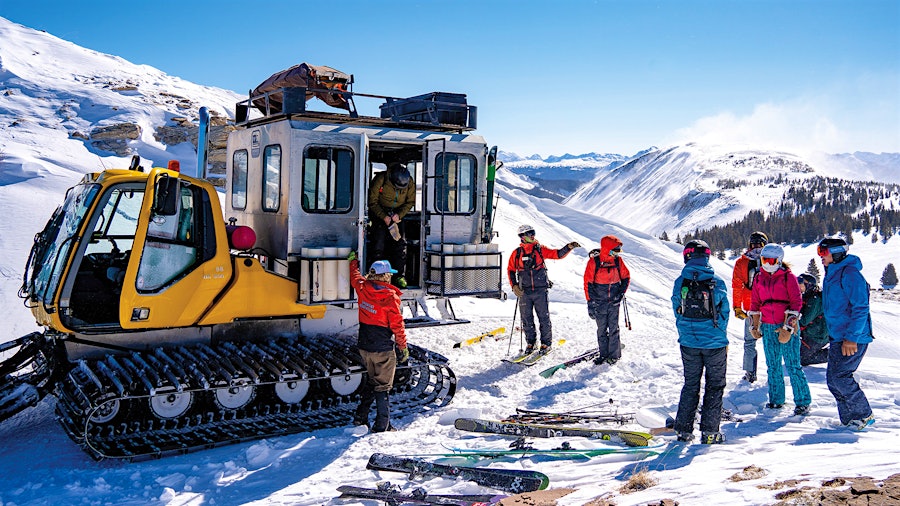This vibrant color photograph captures a picturesque scene at the top of a snow-covered mountain, under a clear blue sky with minimal clouds. Dominating the background is a majestic mountain range, with evergreen trees dotting the landscape. In the right-hand portion of the image, a group of seven skiers, clad in a coordinated red and blue color scheme, stands in the snow, preparing for descent. They are bundled up in winter jackets, long leggings, ski helmets, hats, and are equipped with ski goggles and masks to shield them from the cold. Most of their skis lie on the ground nearby.

To the left, a distinctive yellow snowcat, a grooming vehicle with treads similar to those of a bulldozer, is parked. This snowcat features an open cab and an attached large gray rectangular cabin with windows and a surrounding fence on top, which holds a bag and a box. One person is seen holding the door open, assisting another individual who appears to be stepping down from the cabin. The scene suggests that the group has just been dropped off by the snowcat and is getting ready for their ski trip down the mountain. In the distance, more snowy peaks stretch towards the horizon, completing this stunning alpine vista.